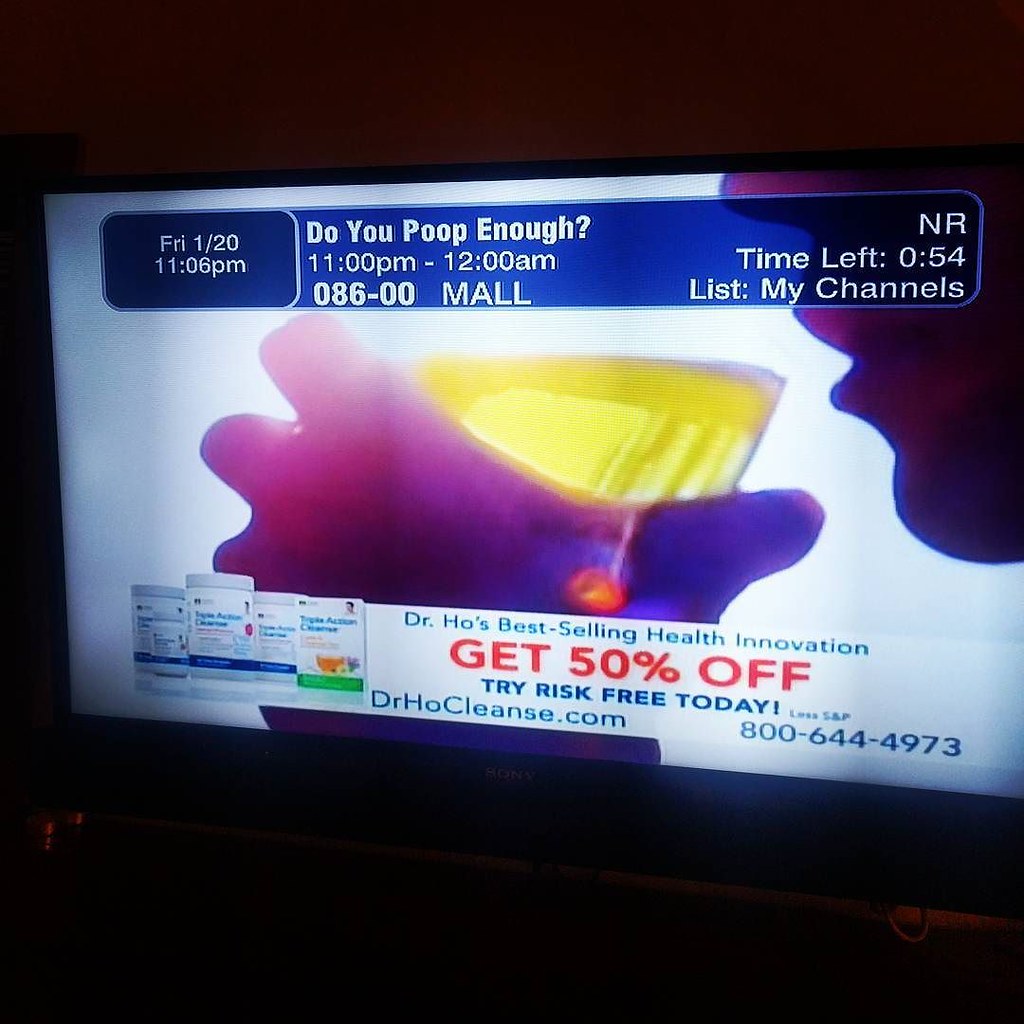The image appears to be a photo taken of a television screen in a dark room, highlighting a late-night infomercial. Across the top of the screen, in white text, it reads "Friday, 1/20, 11:06 PM." To the right, it asks, "Do you poop enough? 11 PM to 12 AM, 086-00 mall." Further right, the display shows "NR, time left 54 seconds, list my channels." The central image features a purple silhouette of a person's face appearing to drink a yellow liquid from a glass. At the bottom, it advertises "Dr. Ho's best-selling health innovation," offering a "50% off, try risk-free today" promotion with the website "drhocleanse.com" and an 800 number. To the left of the bottom section, there are images of pill bottles related to the advertised product.